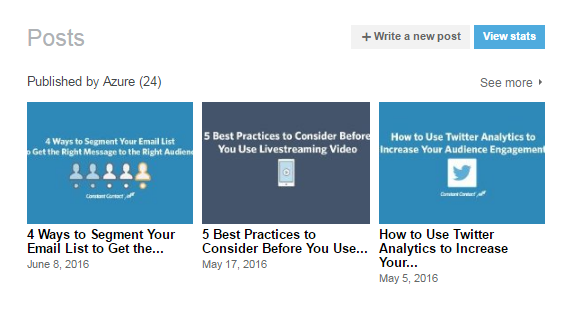This is a close-up screenshot of a website interface. In the top left corner, there is a label in light grey color that says "Posts." On the top right, there are two tabs: one with a plus sign that says "Write a new post" and another blue tab labeled "View stats." Beneath this header, on the left side, it reads "Published by Azure" with the number 24 in brackets next to it, while the far right features a "more" option.

Under this section, there are three rectangular images aligned horizontally. The images on the left and right have a light blue background, while the one in the middle has a very dark blue background. 

The first image on the far left is titled "Four ways to segment your email list and get the right message to the right audience," accompanied by an illustration of five small human figures. This post is dated June 8, 2016.

The middle image is titled "Five best practices to consider before you use live streaming video," featuring a picture of a cell phone. The post is dated May 17, 2016.

The image on the far right is titled "How to use Twitter analytics to increase your audience engagement," with an image of the Twitter logo. This post is dated May 5, 2016.